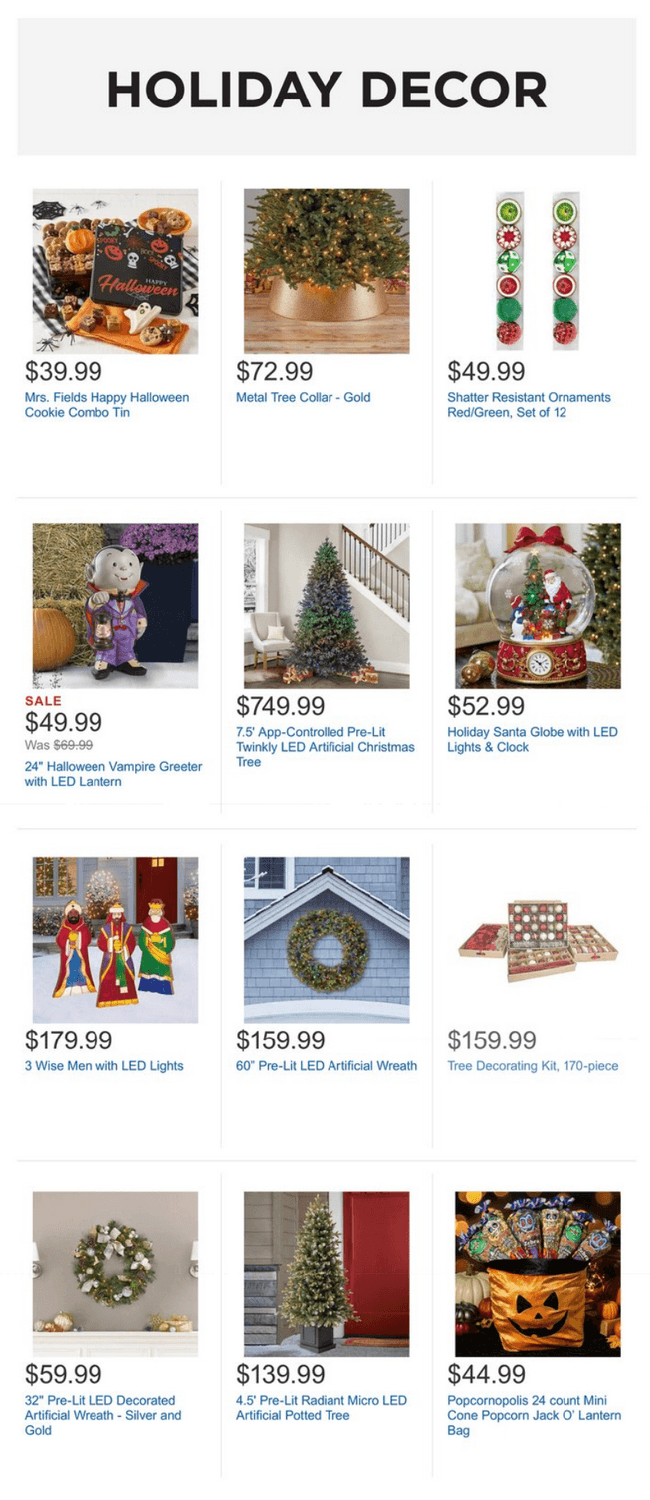The image depicts a web search results page dedicated to holiday decor. Across the top, a gray banner prominently displays the phrase "Holiday Decor" in a black font. Various items related to holiday decorations populate the search results below.

1. The first item is a Mrs. Fields Happy Halloween Cookie Combo Tin, priced at $39.99. This Halloween-themed decor item features an assortment of festive cookies.
2. Next, a gold tree collar is listed at $72.99, offering a stylish base for a Christmas tree.
3. For $49.99, a set of 12 shatter-resistant ornaments in red and green is available for purchase, perfect for adding a traditional touch to holiday decor.
4. Also priced at $49.99, there is a 24-inch Halloween greeter in the form of a vampire, ideal for welcoming guests with a spooky flair.
5. A 7.5-foot LED artificial Christmas tree is available for $749.99, providing a grand and illuminated centerpiece for holiday celebrations.
6. A holiday Santa snow globe featuring LED lights is listed for $52.99, capturing quintessential holiday charm.
7. Finally, for $179.99, a set of three wise men with LED lights is offered, adding a classic nativity scene element to the decor options.

Each item is vividly described in the search results, inviting viewers to explore these festive decoration choices in detail.